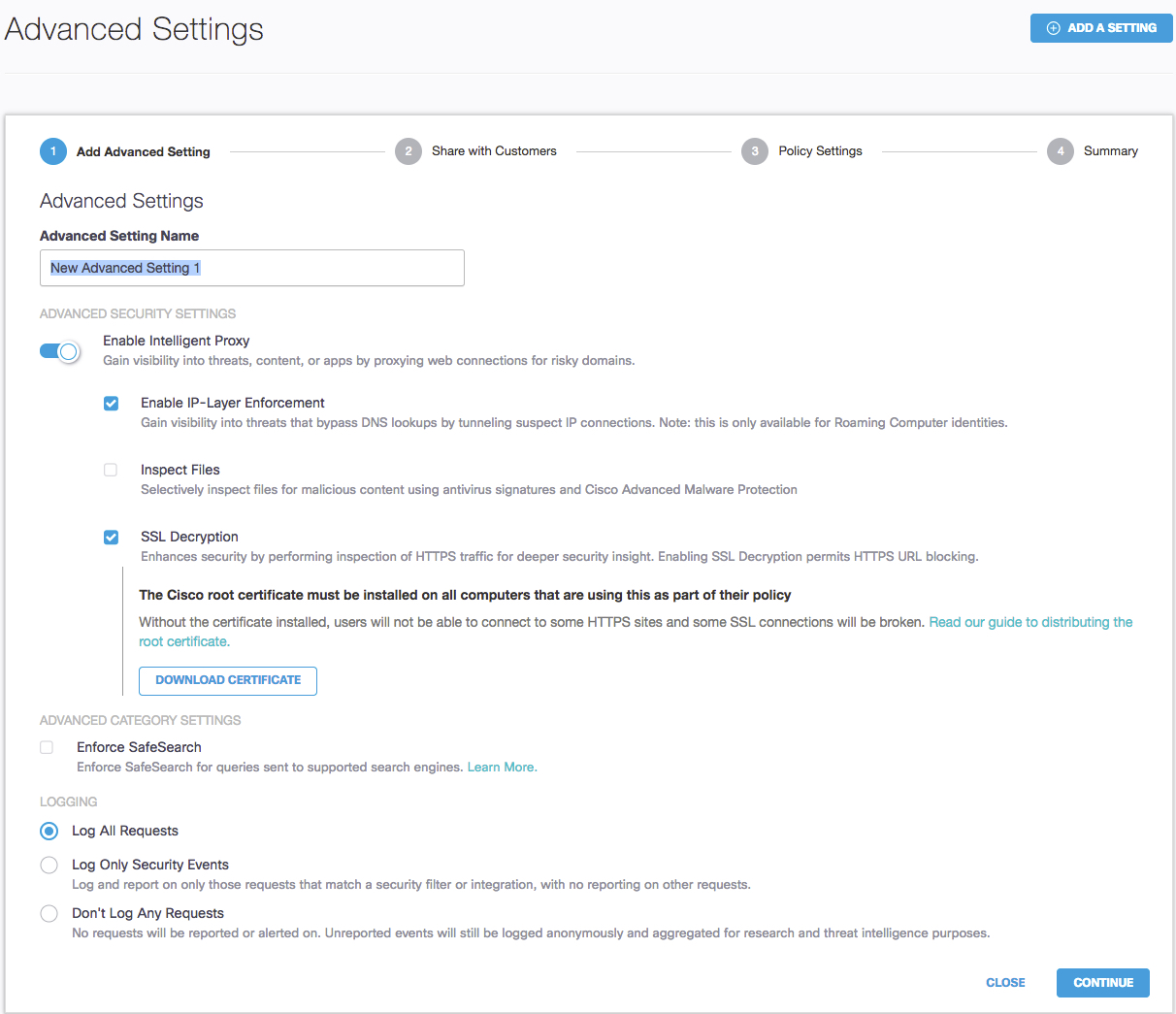The image depicts a user interface for advanced settings configuration:

- At the top left, the text "Advanced Settings" is displayed in black.
- On the top right, there is a blue button labeled "Add a Setting" with white text and a blue plus icon.
- A large white box encapsulates most of the image's content.

Within this box:
- At the top, a number "1" is encircled in blue, accompanied by the text "Add Advanced Setting."
- The numbers "2. Share with Customers," "3. Policy Settings," and "4. Summary" are listed below but are grayed out.

- Under "Add Advanced Setting," the text "Advanced Settings" appears again.

- Below this, there is a labeled box for entering an "Advanced Setting Name."

- Inside this box, "New Advanced Settings 1" is highlighted.

- Below, there's a section titled "Advanced Security Settings," featuring several options:

  - A slider bar labeled "Enable Intelligent Proxies" (currently on).
  - Checkboxes for "Enable IP Layer Enforcement" (checked), "Inspect Files" (unchecked), and "SSL Decryption" (checked).

- Below these checkboxes is a small white button with blue text reading "Download Certificate" and grayed-out text "Advanced Category Settings."

- An additional checkbox is labeled "Enforce Safe Search."
  
- The "Logging" section follows, with three radio button options:
  - "Log All Requests" (selected)
  - "Log Only Security Events"
  - "Don't Log Any Requests"

- In the bottom right corner, two buttons are present:
  - A white button with blue text that says "Close."
  - A blue button with white text that says "Continue."